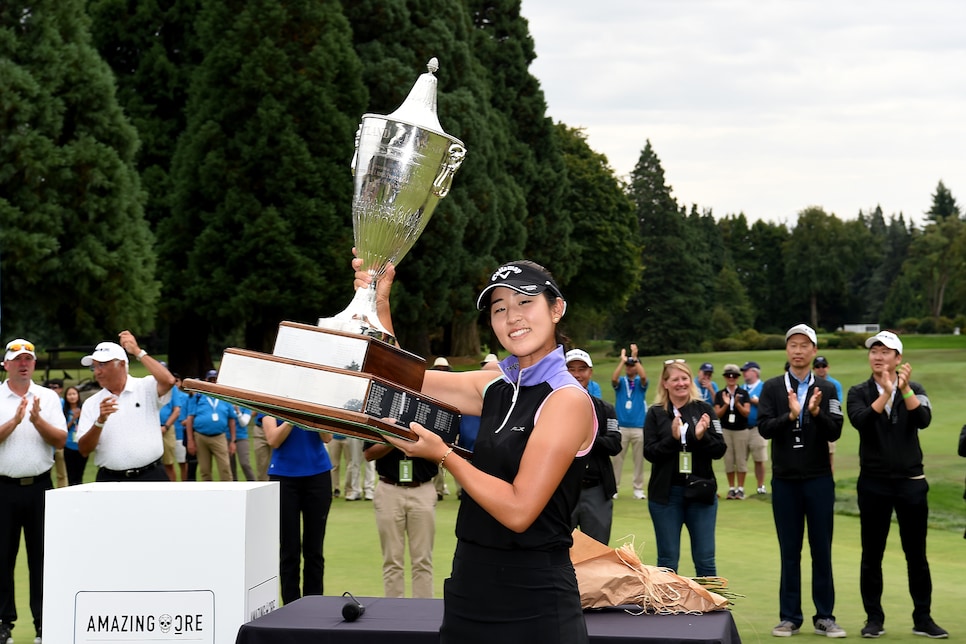In this photograph, a young Asian woman in her 20s, dressed in a black and purple outfit with a black baseball cap, stands proudly on the green of a golf course, holding a large silver trophy that is nearly as big as she is. A bracelet adorns her left wrist. In the background, a mix of players and staff can be seen clapping in her honor. Among them, some are dressed in black outfits, and others in blue polo shirts, all wearing employee press badges on lanyards around their necks. A few older individuals in the right-hand side of the image are wearing white shirts and hats. The backdrop features a serene line of pine trees under clear gray skies. On the lower left of the photograph, a white box with the words "Amazing Ore" can be seen along with a black table displaying various objects. The setting exudes the celebratory atmosphere of a golf club event, possibly capturing a significant win.